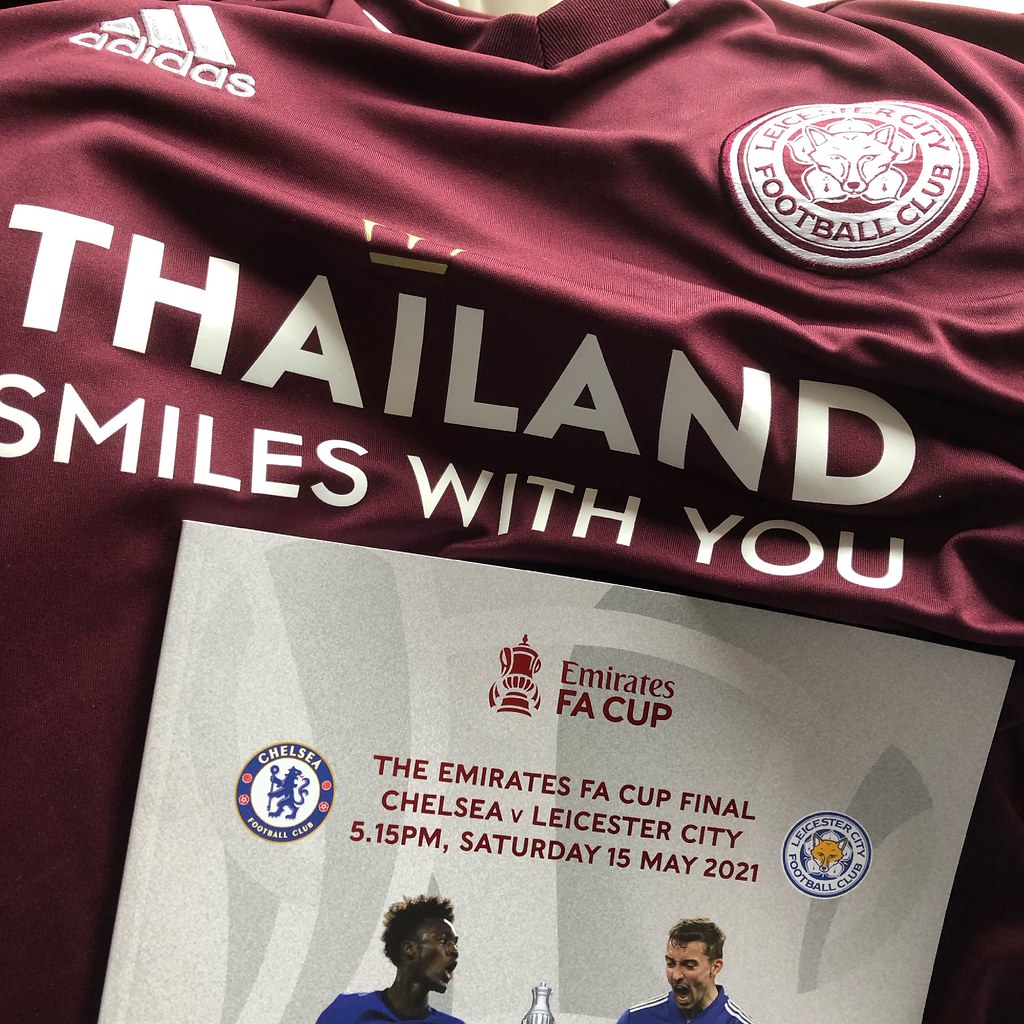The photograph features a maroon Adidas t-shirt, prominently displaying the Adidas logo in the upper left corner and the Leicester City Football Club logo in the upper right corner. Bold white text spans across the chest, reading "Thailand Smiles With You." A white cardstock (placard) is placed on the t-shirt, headlined with "Emirates FA Cup" next to the Emirates FA Cup logo. Below this, the text announces the Emirates FA Cup Final: Chelsea vs. Leicester City, scheduled for 5:15 p.m. on Saturday, May 15, 2021. The logos of Chelsea (a lion holding a spear) and Leicester City Football Club are also featured on this placard. The bottom portion of the photograph includes two men, one appearing to be African and dressed in a blue shirt, and the other a white male in a blue jacket with white stripes down the shoulders.